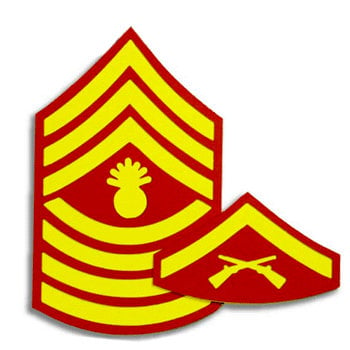The image displays two military-themed patches against a white background. Both patches are predominantly red and have yellow designs. The smaller patch, which is positioned to the lower right, is in the shape of a triangle with a rounded bottom. It features a single blue stripe that extends to a point, above which two yellow rifles are crossed in an X formation, depicted in outline form. This patch is approximately one-third the size of the larger patch.

The larger patch, situated to the upper left, has a distinctive shape with three pointed chevron stripes on the top and three semi-circular chevrons on the bottom, creating a curved edge. Seven yellow stripes in total set against the red background form the intricate design of this patch. The center of this larger patch is decorated with a yellow pineapple shape, detailed to give the impression of a fruit with a textured surface and a leafy crown at the top. The elements of rank and insignia on these patches suggest a military designation or status symbol, possibly suited for a coat or uniform.